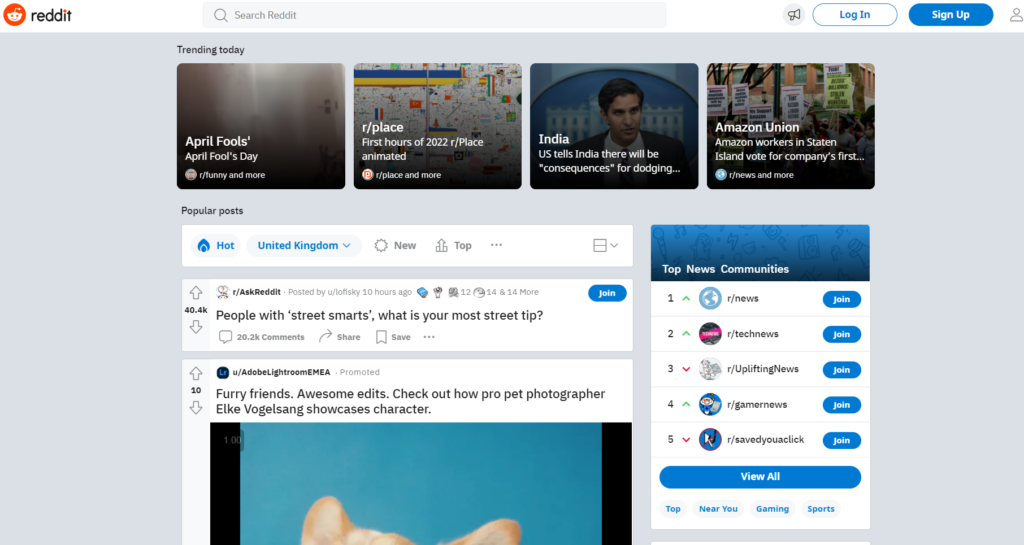### Detailed Descriptive Caption for Reddit Homepage Image:

The image captures Reddit's homepage featuring a distinct layout characterized by a white and light blue color scheme. Across the top border, approximately a quarter-inch bottom border is white, transitioning into a light blue background extending down to the bottom of the screen. On the upper left corner, Reddit's iconic logo is prominently displayed — a red circle encompassing a white robot, adjacent to the black text 'reddit' with the dot above the 'i' colored red.

Beside the logo, there's a search bar with 'Search Reddit' written in black text on a light blue background. About an inch to the right, a light blue circle containing a horn-like signal icon is present. Next to this, there are two buttons: one outlined in blue with a white interior labeled 'Log In' in blue text, and the other a solid blue button reading 'Sign Up' in white text. To the far right, a player or person icon is visible.

The light blue section also features an inch-wide margin on both the left and right sides. Towards the top left, the header 'Trending Today' is displayed, under which four images are arranged. The first image is labeled 'April Fool' and features a red border. The second image, titled 'Reddit/r/place', is a map-like graphic. The third image shows a man with dark hair against a blue background, representing the 'India Amazon Union'. In this picture, people are seen outside holding signs. Beneath these images, a brief description accompanies each.

On the left side of the page under the trending section, a 'Popular Posts' header is followed by a white tab labeled 'Hot' and another marked 'United Kingdom'. Below these, a sequence of Reddit posts is displayed with a small visual preview. One of these posts features an image extending off the bottom of the screen.

To the right of the posts, a blue bordered area roughly an inch wide features the header 'Top New Communities.' This section lists five communities beneath it, each represented with their respective icons. A blue tab labeled 'View All' in white text spans the width under the community list. Further below, additional headers read 'Top', 'Near You', 'Gaming', and 'Sports' arranged from left to right, contributing to a well-organized and informative homepage.